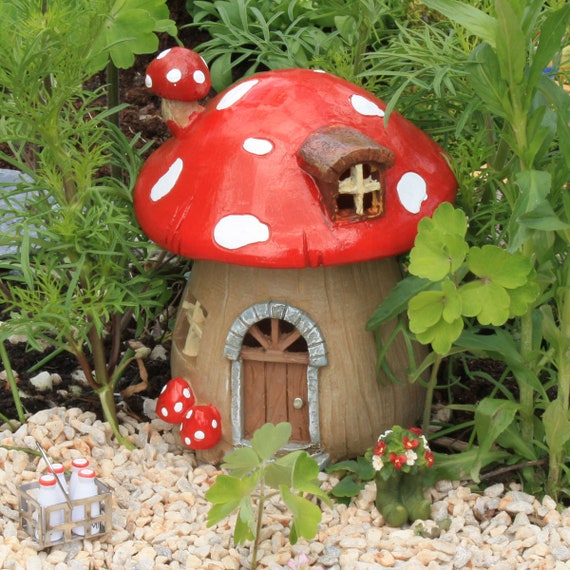This whimsical outdoor photograph showcases a miniature fairy house designed to resemble a toadstool, forming the focal point of the image. The fairy house, positioned centrally, features a light brown stem and a distinctive red cap adorned with white spots, mimicking the appearance of a classic toadstool. The structure includes a quaint wooden door with a gray arch and a small doorknob, nestled amidst a gravel base and surrounded by an assortment of greenery.

To the right of the door stands a potted plant bearing red and white flowers, while to the left, a crate containing four milk bottles with red caps is subtly placed. The top of the house is accentuated with a small attic window and a tiny toadstool sprouting from the larger cap. Encircling the fairy house are diverse plants, creating a lush, leafy backdrop that adds to the enchanting atmosphere. In the foreground, a collection of white pebbles and additional smaller red and white toadstools enhance the scene's fairy-tale charm.